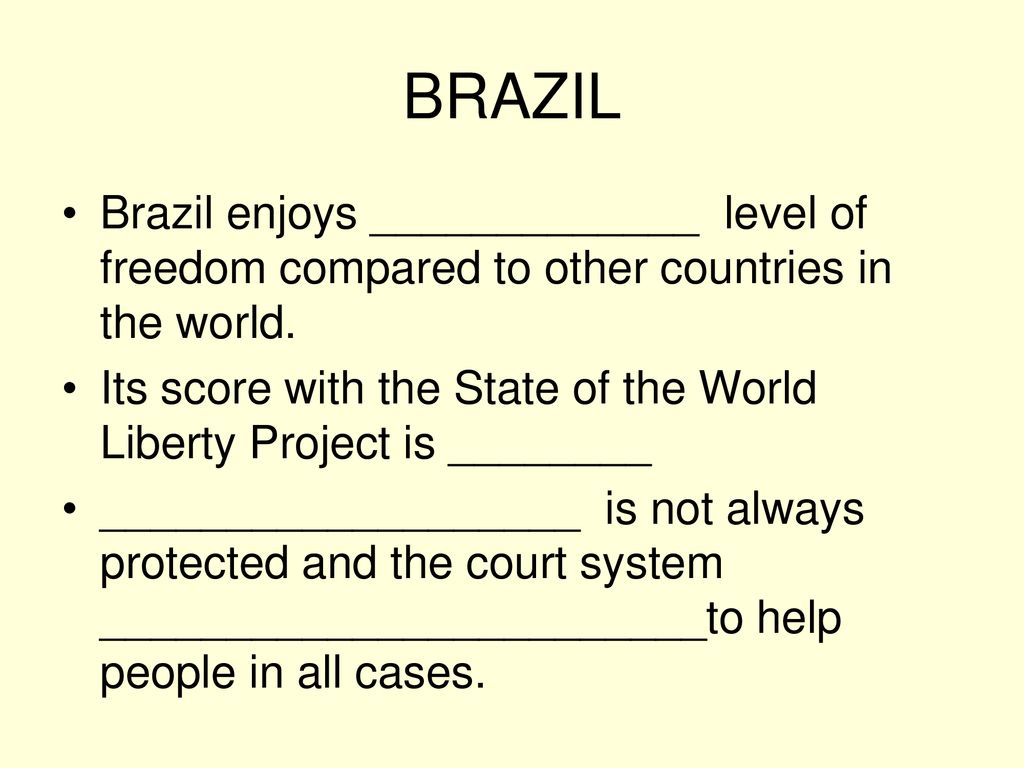This screenshot captures a fill-in-the-blank word puzzle from an article, possibly focusing on freedom and rights in Brazil. The entire page features a light tan background with black text that is organized into three bullet points under the heading "Brazil." The first bullet point reads, "Brazil enjoys __________ level of freedom compared to other countries in the world," with a long blank line indicating where the missing word should be filled in. The second bullet point states, "Its score with the State of the World Liberty Project is __________," again with a long blank line for the score. The third bullet point mentions, "__________ rights are not always protected in the court system, __________ to help people in all cases," requiring fill-ins for two specific terms. This word puzzle seems to invite readers to engage with the content by filling in the appropriate words, presumably based on their knowledge or further research about Brazil's level of freedom, its World Liberty Project score, and the state of rights protection in its judicial system.